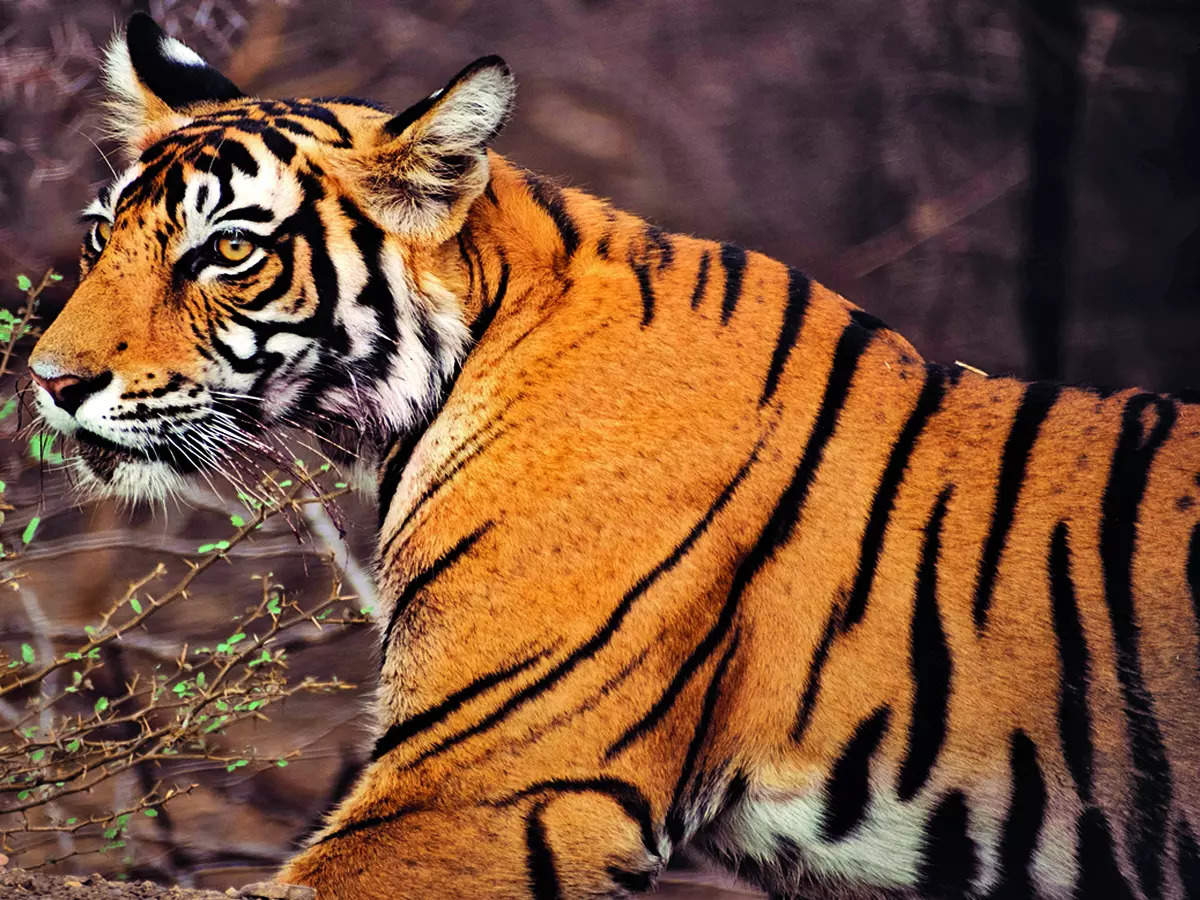The image shows a close-up profile of a large Bengal tiger, positioned sideways with its head turned slightly to the left. The tiger's striking orange fur, adorned with distinctive black stripes, covers much of its torso, shoulders, and head. The face, particularly around the cheeks, chin, and inside the ears, features prominent white fur, contrasting with the orange that dominates its nose and the bridge area. The visible eye, colored a vibrant orange-yellow, catches the light, while only a hint of the other eye can be seen due to the tiger's posture. 

The background is an outdoor scene rendered in blurred hues of brownish-purple, creating a soft, almost chilly ambiance. On the left side of the photo, a few slender tree branches with budding green leaves add a touch of vibrancy to the scene. The tiger's underside, including its belly and part of its back legs, is visible but the paws remain out of frame. The overall effect is a detailed and majestic portrayal of the tiger, accentuated by the contrasting colors and natural setting.